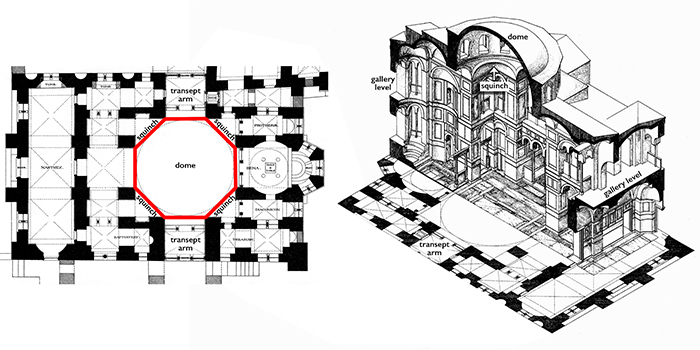This image features a detailed black and white architectural drawing of a large building, possibly a mansion or a museum. It consists of two separate diagrams. On the left, a floor plan highlights various rooms, including rectangular, square, and half-semi-circle formations. A central octagonal area, marked with a red circle, is labeled "Dome," with each corner labeled "Squinch." Adjacent to the Dome, two areas are marked "Transept Arm." 

The right-hand side displays a 3D cross-sectional sketch of the building, revealing a tall structure with multiple stories. This cross-section also labels the "Dome" at the top and "Squinch" beneath it. A level termed "Gallery Level" is noted, corresponding to an exhibition or significant room within the building. The Transept Arm is also marked towards the bottom, serving as a key connector between different sections of the structure. The detailed annotations across both diagrams help in understanding the spatial arrangement and functional divisions of this museum-like building.